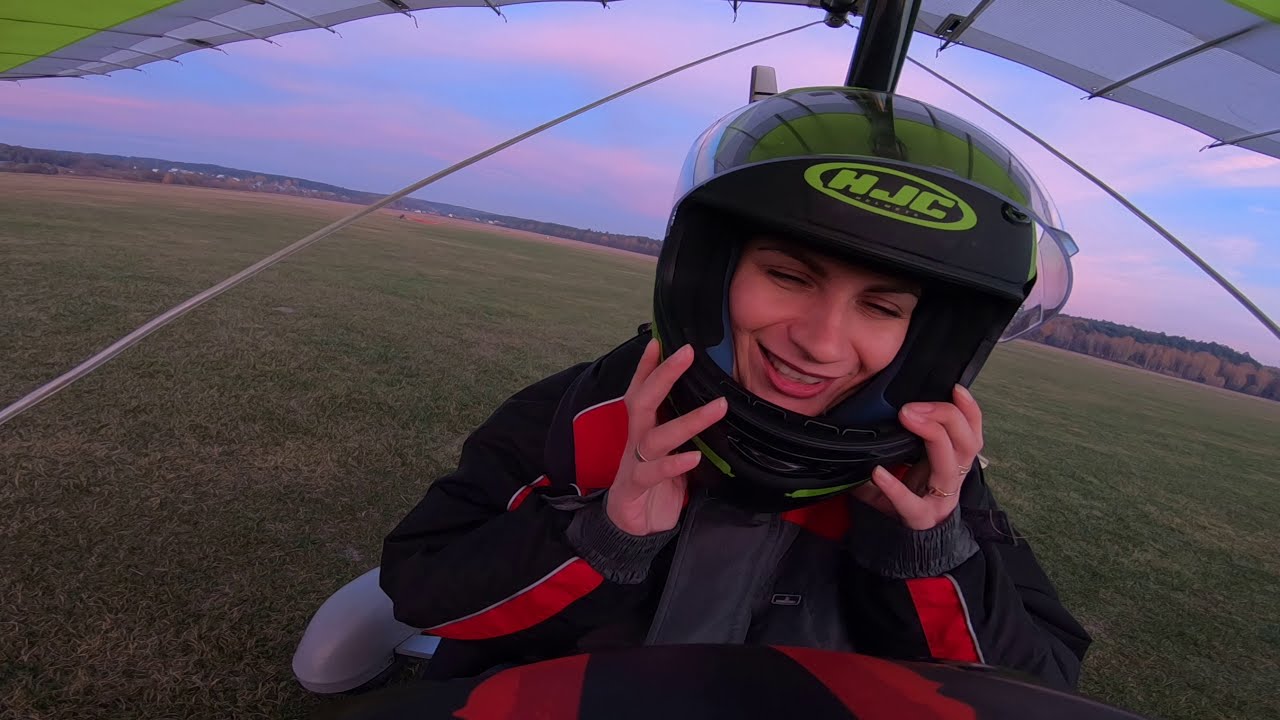In this color landscape photograph, a young white woman in her 20s is the focal point, captured up close and looking down with a smile. She is wearing a black helmet with a bold neon green "HJC" graphic on the front, and a black jacket highlighted with red and white stripes on the sleeves. Numerous rings adorn her hands, which are raised to touch the sides of her helmet, showing off her manicured nails. She is securely strapped into a hang glider, the yellow and white wings of which are visible extending from the top left to the top right corners of the image.

The setting below her is a green grassy field, stretching across the frame. Although it's challenging to discern whether she is airborne or has just landed, the perspective suggests she might be flying at a very low altitude. In the distance, the horizon features a shallow line of hills with scattered trees and a few buildings, merging into a streaky, hazy blue sky tinged with pink clouds, indicating the soft lighting of near sunset. The photograph presents a realistic and representational depiction of the serene and thrilling moment.